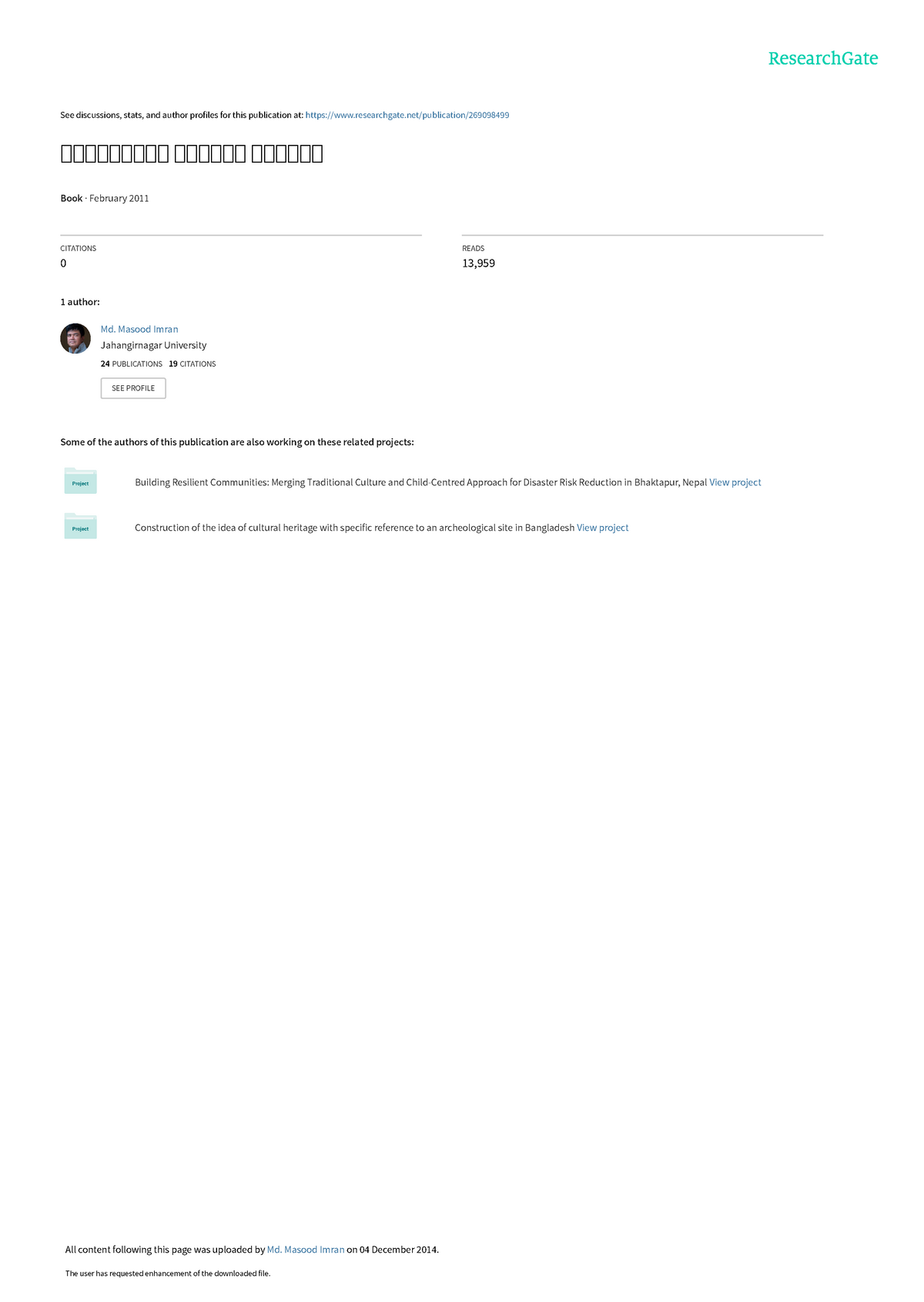This image showcases a publication listing from ResearchGate, an academic platform for sharing research outputs. The image has a white background and is horizontally oriented. In the upper right-hand corner, the ResearchGate logo is displayed in light teal. This platform allows academics to post various types of research including journal articles, book chapters, and manuscripts, aiming to facilitate sharing and feedback rather than formal publication credit.

At the top of the listing, there's a note encouraging viewers to "See discussion stats and author profiles for this publication at" followed by a URL. The centerpiece of the listing is a book published in February 2011, which, despite being 13 years old, has garnered notable attention with 13,959 reads but zero citations. The sole author of this book is Md Massoud Imran from JAHANGIMAGAR University. His profile indicates he has 24 publications and 19 citations to his name. A circular thumbnail image of the author and a button to view his profile are also included.

At the bottom of the listing, there's an update mentioning that some authors involved with this publication are currently engaged in related anthropology projects, hinting at broader academic connections and ongoing research in similar fields.